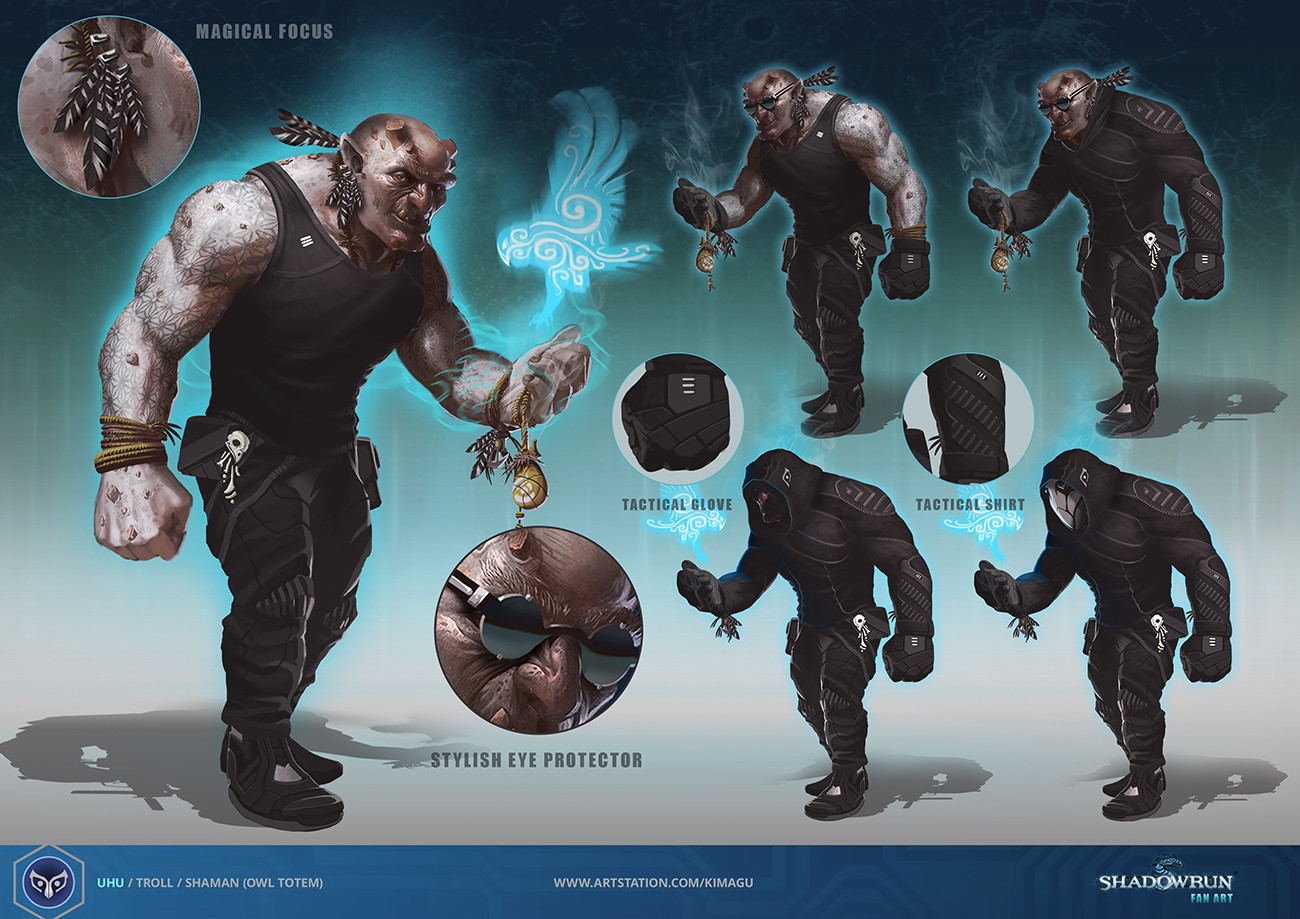This image appears to be concept art for a game, possibly fan art for "Shadowrun," created by the artist at www.artstation.com/kimagu. The central character is a grotesque and muscular troll or shaman with grayish skin and horns that appear to be sawed off. He is depicted wearing a black tank top, black pants, and a fanny pack adorned with small skulls, indicating a dark or mystical character. The character on the left is the primary focus, standing confidently with an eerie, spectral owl floating above his outstretched hand, symbolizing his magical abilities.

To the right, there are four smaller versions of this character, each showcasing different outfits and accessories. Some wear tactical shirts, gloves, and masks, including one that resembles a beak, while others sport stylish eye protection, likely a pair of glasses. These attire variations suggest different roles or classes within the game, enhancing the character's versatility. Alongside the different attires, one can see descriptions like "tactical glove," "tactical shirt," and notably, an "earring of feathers."

At the bottom of the image, a dark to light gradient bar contains pertinent information. It reads "U-H-U / troll / shaman (owl totem)" and "Shadowrun fan art," supporting the theme of the artwork. This detailed illustration underscores the character's complexity and the rich, imaginative world he inhabits.